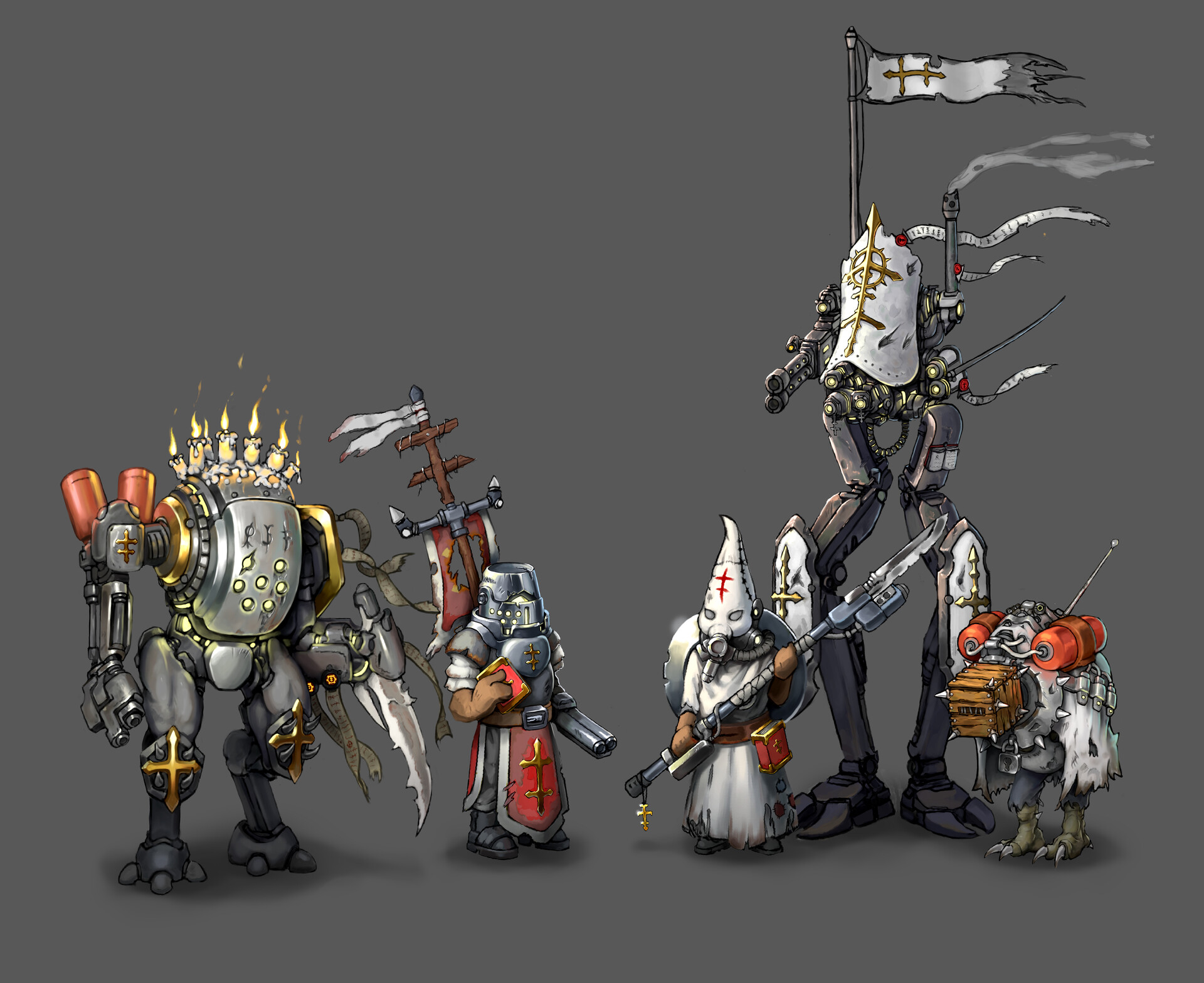The image is set against an all-gray background with darker gray shadows beneath the characters, adding depth. There are three primary figures, each appearing as if they belong in a comic, animated movie, or video game, with distinctive and highly detailed appearances.

On the far left is a character that looks like a silver and gray robotic creature with a distinct steampunk aesthetic. This robot has lit, melting white and yellow candles on its head, with golden crosses adorning its knees. Its left arm ends in a large, insect-like blade and its left shoulder features a red canister, while its right hand wields guns and knives.

Next to it stands a more humanoid figure clad in a mix of armor and a red skirt. This character has a double-barrel shotgun for a left hand, carries a flag with red and white symbols, and has a cross emblem on its chest and lower parts. The lights embedded in the helmet are yellow, and the outfit consists of gray pants and boots. The character holds a red and yellow book in the right hand.

On the right is a figure draped in a white hooded outfit reminiscent of a Ku Klux Klan hood but with a gray gas mask covering the face. The hood features a red cross painted on it, and the character wields a long bladed weapon on a stick. This character is in an all-white gown and carries a red and gold book in the left hand.

Overall, these characters are vibrant and distinct, each with a unique blend of armor, weaponry, and symbolic features, set against a stark backdrop that highlights their detailed designs.